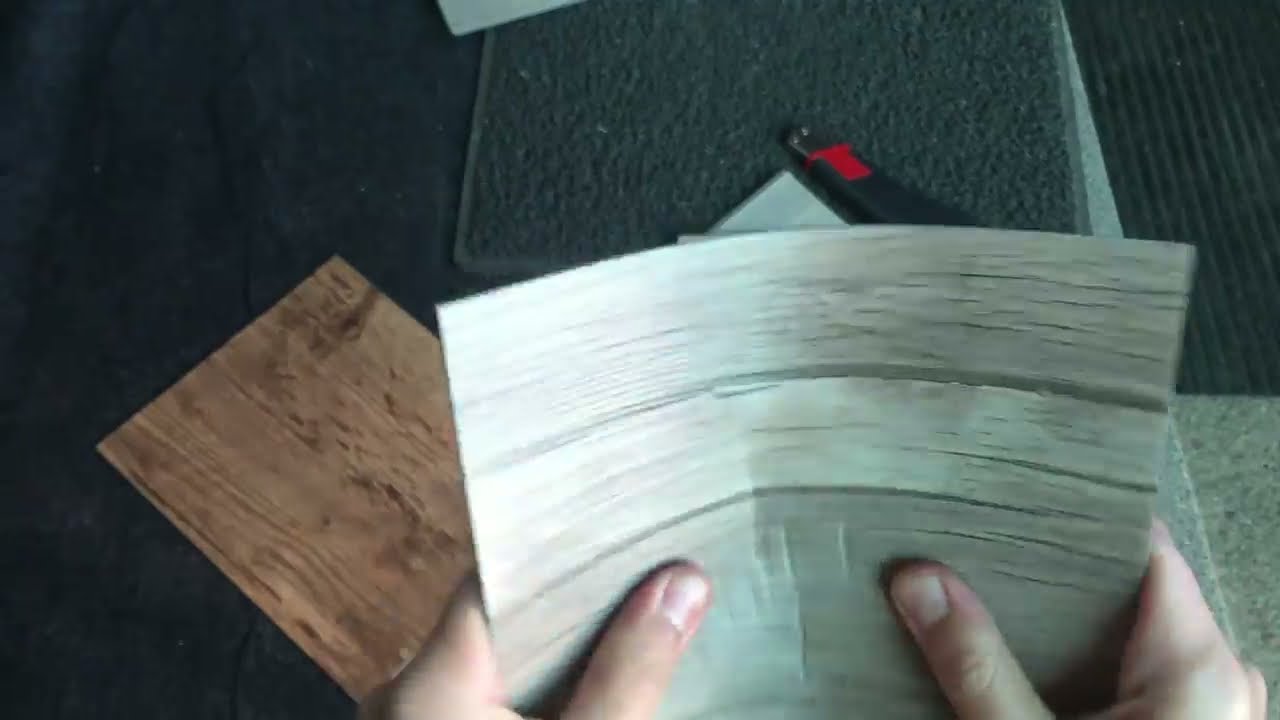In the detailed close-up image, we observe a meticulous floor renovation project. The setting features a variety of wood-grained tile samples placed on a speckled gray concrete surface, indicative of a workspace. Visible at the bottom middle of the image, three fingertips are engaged in the task, positioned on a wood-grained tile sample. Above the hand, several other tile samples are arranged, showcasing a spectrum of wood tones, including medium wood, gray-washed wood, and light-washed wood. To the left, a darker gray felt piece is noticeable. In the upper middle section, a gray textured mat is present, upon which rests a distinctive red and black retractable utility knife, clearly intended for cutting the materials. The right third of the image displays an active section of the project, where the floor tiles are being adhered to the surface, contrasting with the already completed two-thirds on the left. A doormat is partially visible at the top, hinting at the completion of the intricate tile-laying process.